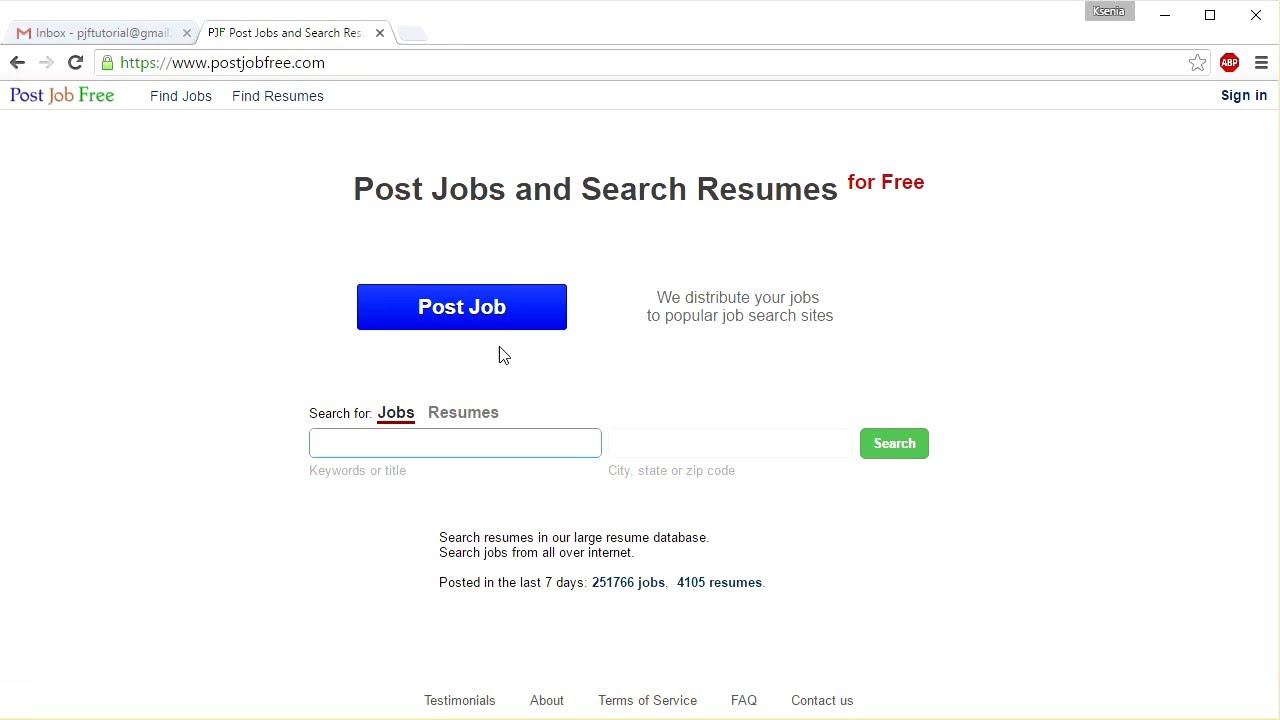Here is a cleaned-up and detailed descriptive caption for the image:

---

The screenshot displays a computer or tablet screen navigating the PostJobFree website. In the top left corner, the word "Inbox" is visible, indicating the active inbox for the email account "PJFTutorial@gmail.com." Next to this, there is a tab labeled "PJF post jobs and search" with a small 'X' next to it for closing the tab.

At the top right corner of the screen, a checkbox labeled "KSEMIA" is present but not checked, followed by an 'X' for closing. Directly beneath this section, within the address bar, there are navigation icons including a left-pointing arrow and a circular arrow, along with a padlock symbol indicating a secure connection. The URL displayed is "https://www.postjobfree.com.”

Below the URL bar, the homepage text reads "Post Job Free. Find jobs, find resumes, sign in." This is followed by a navigation bar stating "Post Jobs and Search Resumes," with the phrase "for free" highlighted in red. A blue rectangle with the "Post Job" button is prominently placed, accompanied by the text "Redistribute your jobs to popular job search sites."

The page then provides a search function featuring an empty text box meant for input. Underneath, there are labels "Keywords or title" and "City, state, or zip code," with an adjacent green rectangular “Search” button. Further descriptions promote the website's offerings with text such as "Search resumes in our large resume database" and "Search jobs from all over the internet." It specifies that there are 251,766 jobs posted in the last seven days and a database containing 4,105 resumes.

---

This caption incorporates all the elements from the verbal description, organizing them coherently and providing a clear, detailed overview of the screenshot.